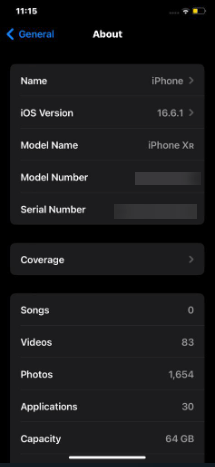The image captures a close-up view of an iPhone screen displaying the "About" section under "General" settings. The upper-left corner shows the current time as 11:15 in white text. The upper-right corner features a Wi-Fi symbol and a battery icon, the latter indicating roughly 40% battery life with a yellow marker within a white outline. Below, the screen heading shows a blue title "General" on the left and a white title "About" on the right, confirming the user is viewing the device's information settings. 

Detailed device information is listed below:
- **Name:** iPhone (white text on the left)
- **Software Version:** iOS 16.61 (white text)
- **Model Name:** iPhone XR (grey text)
- **Model Number:** Obfuscated by a grey box
- **Serial Number:** Obfuscated

Next, a new section details content and capacity:
- **Coverage:** [Details not specified]
- **Songs:** 0
- **Videos:** 83
- **Photos:** 1,654
- **Applications:** 30
- **Capacity:** 64 GB

This thorough depiction of settings and statistics gives a comprehensive overview of the device's status and storage usage.